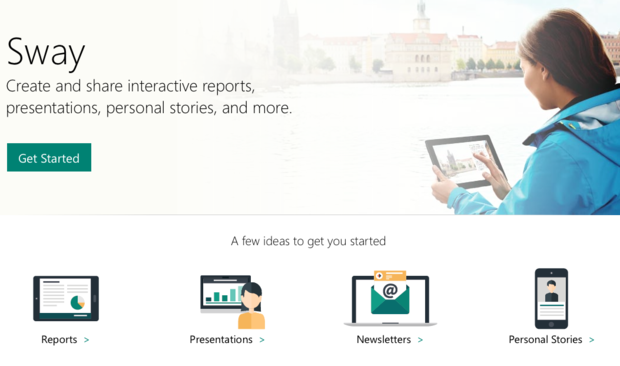This cropped screenshot portrays the interface of the Microsoft Sway app, a tool designed for creating reports, presentations, and social media content. At the top of the image, there is a photo background of a woman crafting a blog post from a picture she has taken of a building across a river. To the left, in bold black letters, is the word "Sway." Below this, the text reads, "Create and share interactive reports, presentations, personal stories, and more." Beneath that message, there is a prominent green "Get Started" button. Centered at the bottom of the screenshot, in small black font, it states, "A few ideas to get you started." Below this text are four thumbnails. The first thumbnail depicts a presentation and is labeled "Reports." The second features a bar graph and is labeled "Presentations." The third shows a newsletter icon and is labeled "Newsletters." The fourth, on the far right, displays a cell phone icon and is labeled "Personal Stories." The remainder of the content is cropped out of the image.